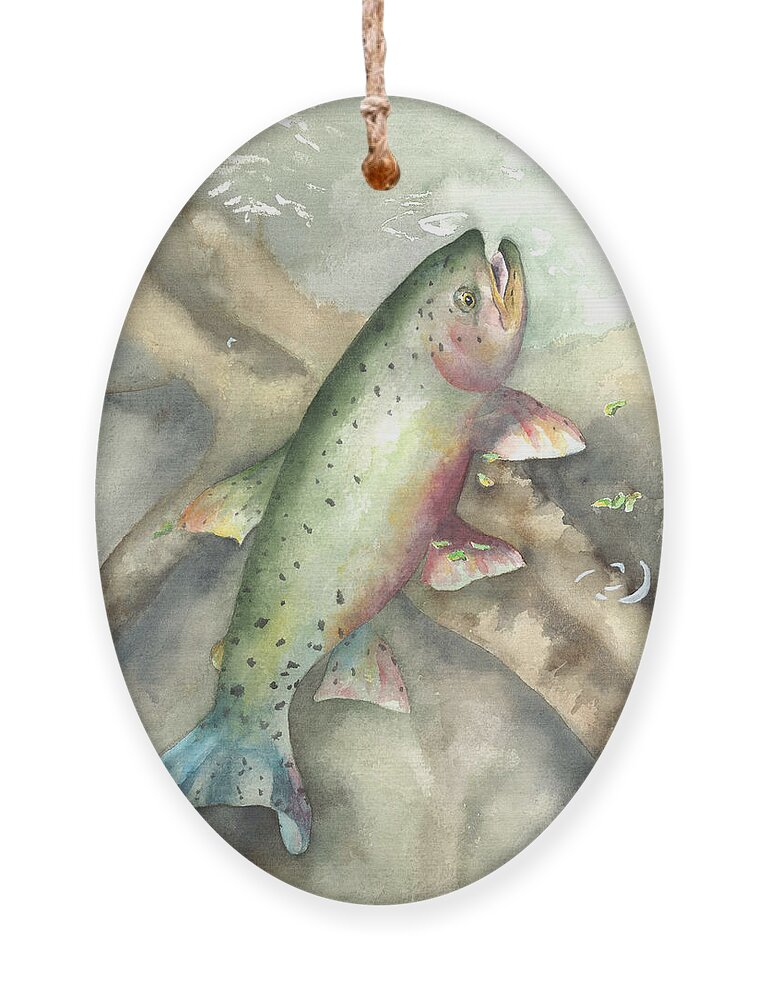This detailed image captures an oval-shaped ornament that combines artistic finesse with versatile usability. It features a hand-painted, multicolored fish, likely a trout, adorned with intricate details that highlight its vivid coloration: a green-speckled back, a bluish tail, and a darker, purple-like belly. Its open mouth and observable eye give the impression of it reaching for food near the surface. The background is a soft watercolor wash of grays and light browns, with an indistinct second fish blurred behind, further emphasizing the primary fish.

The ornament, which could be year-round decor, has a hole at the top with a cord threaded through it, suitable for hanging on a Christmas tree, a window with a suction cup, or from a door handle. The pendant's size is indeterminate from the image, leaving it ambiguous whether it’s meant for a wall hanging, necklace, or some other use. The colors predominately feature a palette of mossy greens and light blues, with touches of reddish hues and brown wood beneath the fish, blending beautifully in a soft, watercolor style.